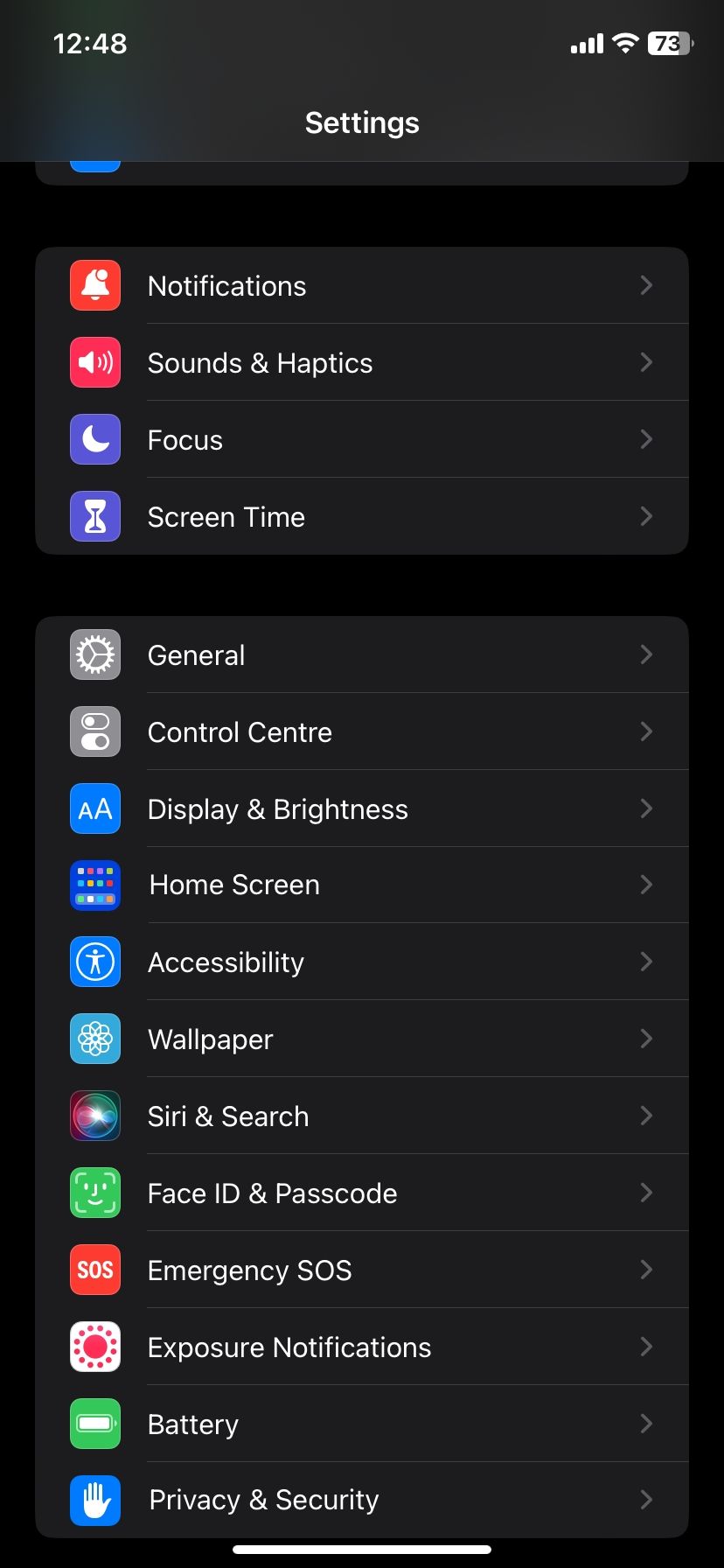The image displays a mobile device screen set against a black background. In the top left corner, "12:48" is displayed alongside four signal bars, a Wi-Fi icon, and a battery symbol indicating 73% charge. Below the status bar, the main heading reads "Settings," followed by a vertical list of settings categories. Each category has an icon on its left and a greater-than symbol (>) on its right. The categories are organized as follows:

1. **Notification**
2. **Sound and Haptics**
3. **Focus**
4. **Screen Time**

Separated by a distinct divider, the next set of categories includes:

5. **General** (represented by a gear icon)
6. **Control Center**
7. **Display and Brightness** (denoted by a blue square with two capital A's inside)
8. **Home Screen**
9. **Accessibility**
10. **Wallpaper**
11. **Siri and Search**
12. **Face ID and Passcode**
13. **Emergency SOS**
14. **Exposure Notification**
15. **Battery**
16. **Privacy and Security**

Each section presents intuitive icons and clear labels, facilitating easy navigation through the settings menu.